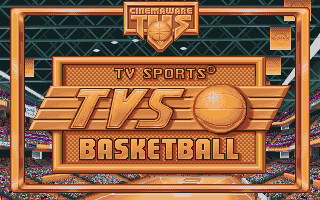This digitally designed graphic features a landscape orientation with a distinctly cartoonish aesthetic. Dominating the foreground, the text "TV Sports" and "TVS Basketball" is prominently displayed on an orangey-brown surface, accompanied by a basketball icon adjacent to the "TVS" letters. The background showcases a computer-generated interior of a basketball stadium, including the court floor in matching orangish-brown hues and three tiers of seating areas. Although individual spectators are indistinct, the scene suggests a populated, lively arena. Crowning the composition, the header "CinemaWare TVS" is prominently positioned at the top.